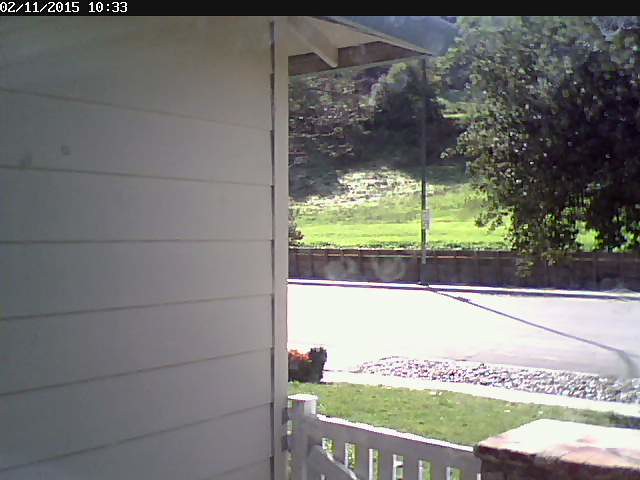This image appears to be a still from a doorbell camera used for property surveillance. Captured on February 11th, 2015 at 10:33 AM, the scene is brightly lit, indicating daylight hours. The frame features a house with white trim and a white fence in the foreground. In the background, there is visible greenery, suggesting a landscaped yard or garden area. Despite the clarity of the surroundings, there is no notable activity taking place in the image, marking it as an uneventful moment in time.